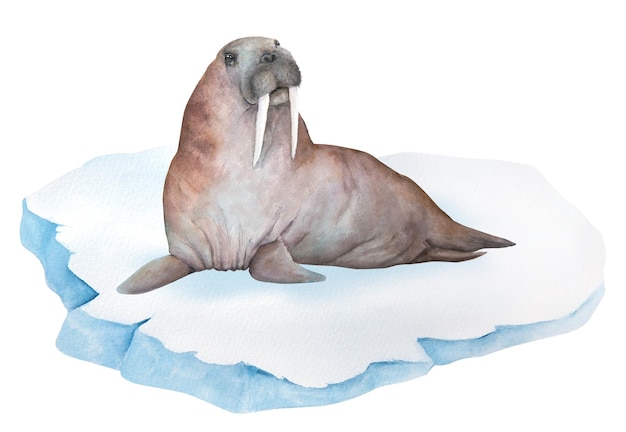In this detailed sketch, we see a large walrus sitting calmly on an irregularly shaped ice floe, set against a white background. The ice is predominantly white with light blue edges, reminiscent of a glacier, and appears slightly wrinkled and broken. The walrus, centrally positioned on the ice, is sketched in a mix of brown and white, with a darker brown on its upper side that tapers to a grayish-brown towards its tail. Its two flippers extend out to the sides, and its small tail is visible at the back. This walrus features long, white ivory tusks hanging down from its mouth, which is slightly open, revealing a large, expressive face with dark eyes, a tiny nose, and prominent folds of skin. The overall illustration is stylized with a blend of realism and cartoon-like elements, giving it a unique character.